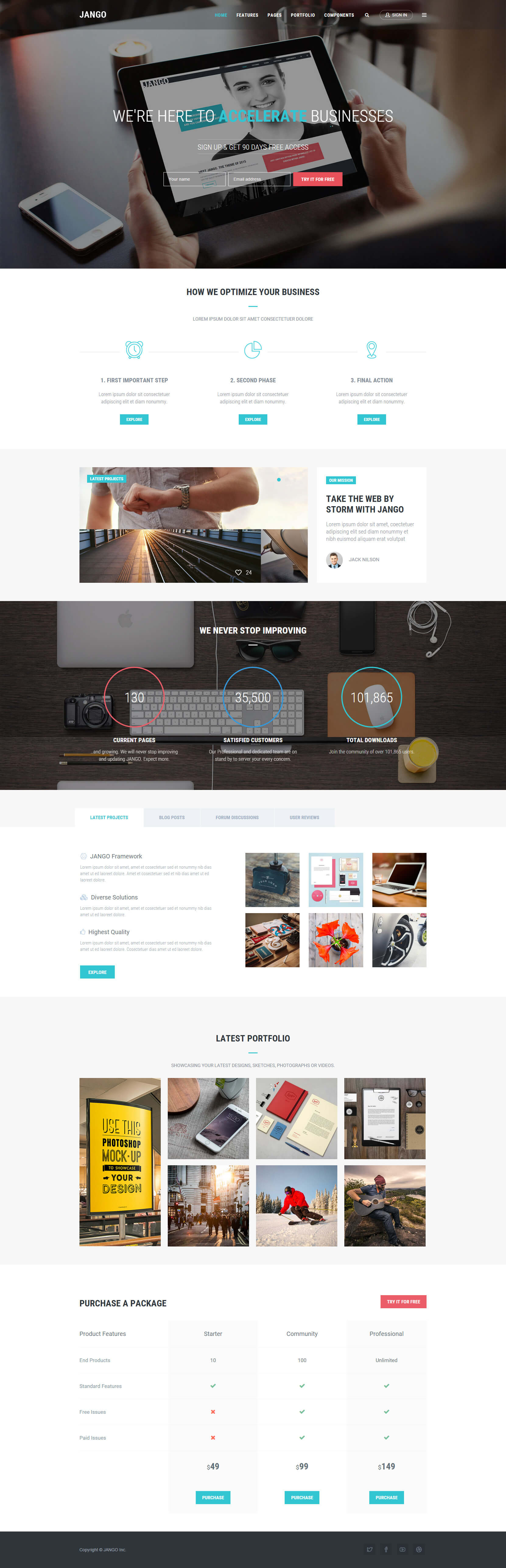The image is a screenshot of a website called Jango, as indicated by the bold "J-A-N-G-O" in the top section. The main feature displayed is a promotional banner showing a person holding a tablet. On the tablet screen, there is a picture of a smiling girl. Overlaid on the banner is a headline that reads "We're here to accelerate businesses," with the word "accelerate" highlighted in teal.

Further down, there is a section titled "How We Optimize Your Business" in black text. This section is divided into three visual steps. The first step is represented by a clock icon labeled "First Important Step." The second step includes a pie graph, and the final step is marked with the number "3" and a map pinpoint icon. Below each step, a teal box with the word "Explore" provides additional information or links for further exploration.

Continuing down the page, the website showcases several images, including one of a keyboard, and features a section labeled "Latest Portfolio." Within this section, the text "We never stop improving" is prominently displayed. Towards the bottom of the page, there is an area titled "Purchase a Package" where users can presumably buy services or products offered by Jango.